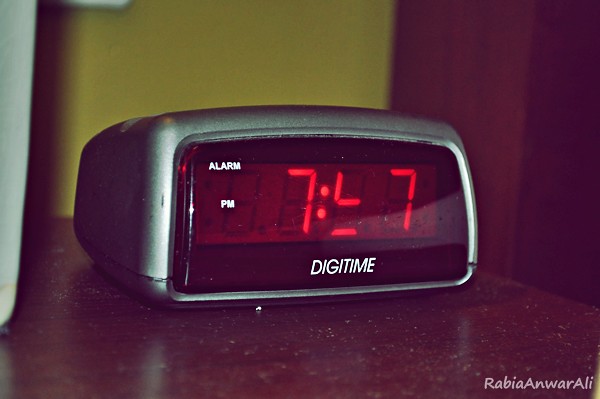This photograph captures a silver digital alarm clock with a rounded rectangular body sitting on a brown wooden surface. The clock's square digital display shows the time as 7:5_7, with the middle digit missing some LEDs, making it unclear whether it’s a five or another number. The time is displayed in bright red text, with "alarm" and "p.m." indicated on the left side of the screen. Below the time, the clock is branded as "Digitime." The background features a yellow wall and a wooden door frame on the right. In the bottom left corner of the image, there is a watermark that reads "Rabia Anwar Ali."